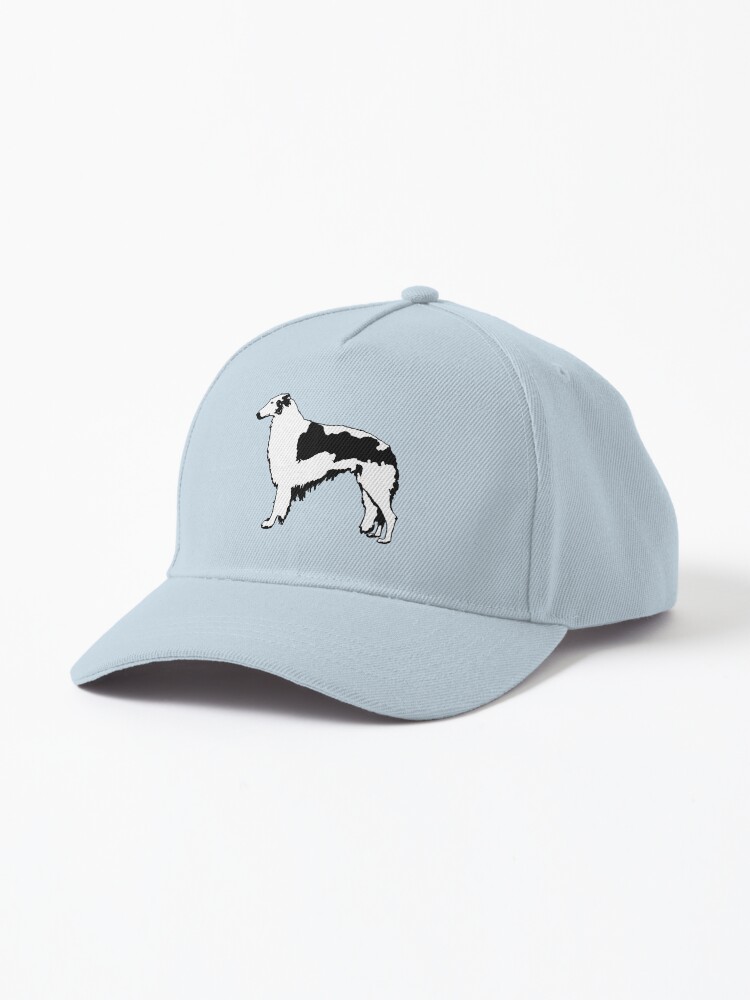This is a detailed photograph of a baby blue baseball cap set against a light gray background. The cap is carefully placed on a white surface, casting a soft shadow to its right, highlighting its three-dimensional form. Distinctly visible on the front of the cap is a meticulously embroidered image of a dog, likely a border collie, characterized by its white body adorned with black patterns. The dog has an elongated face with a narrow snout, black ears, and a notable black patch extending from its shoulders down to its front leg. The six-panel construction of the cap includes a button at the top, and the brim is slightly curved, angling toward the lower left corner of the rectangular photo. This detailed portrayal emphasizes the craftsmanship of both the cap and the embroidered canine image, possibly suggesting it as merchandise related to dog enthusiasts or professional breeders.